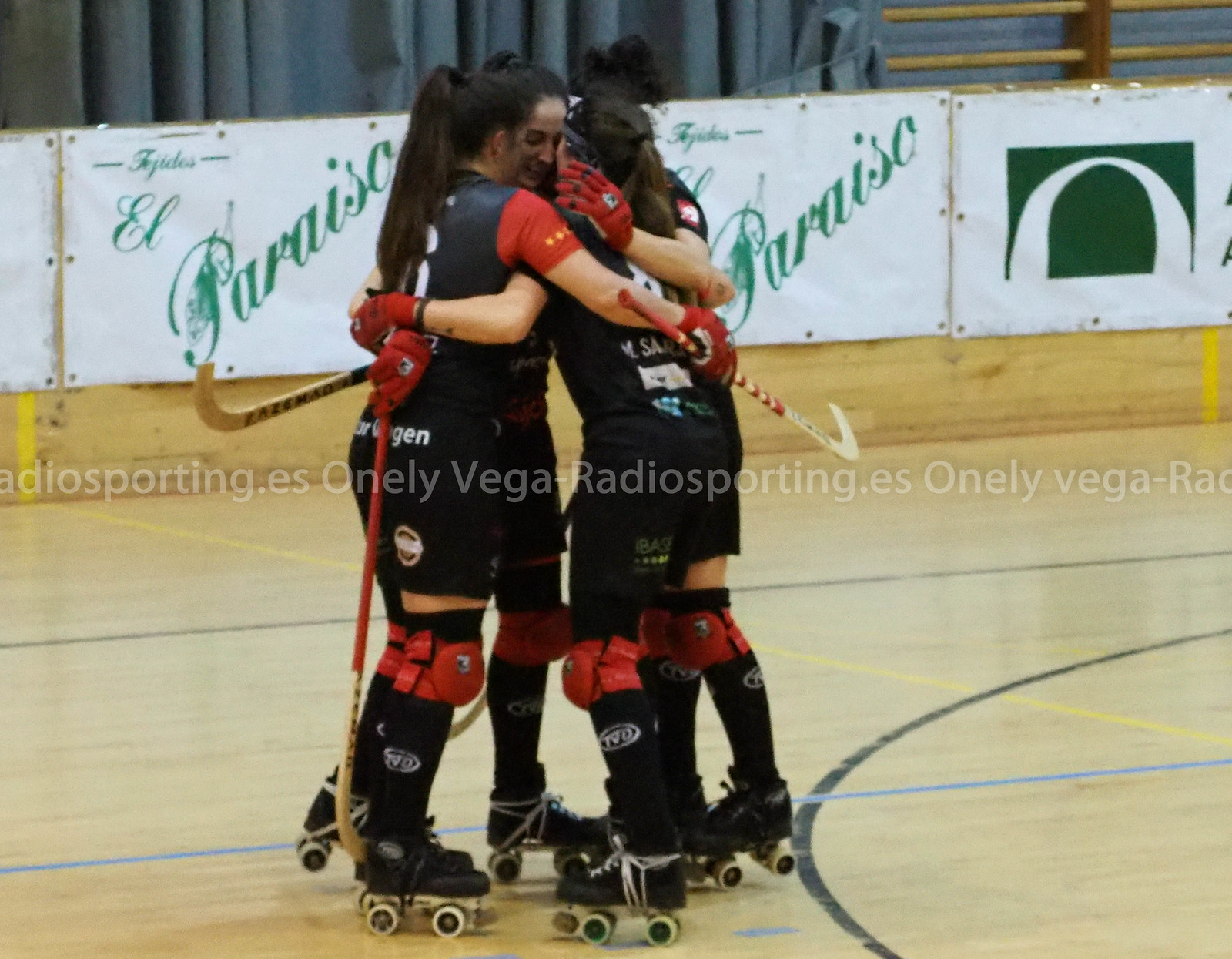This vibrant digital photograph captures three young women in a joyful triple hug on a repurposed basketball court, now a gymnasium floor. They are wearing black hockey uniforms with vivid red knee pads and gloves, all while balancing on roller skates. Each woman holds a hockey stick in one hand, and embraces the others with her free arm. Under their black tank tops, some wear red or additional black shirts. The roller skates are predominantly black, complemented by black socks adorned with a light gray logo. The gym, which exhibits a shiny, light-colored wooden floor, features a partially legible banner in the background with a hint of green, possibly referencing "Parisia" and a European location, suggested by an obscured website address. The background also includes colorful elements in red, yellow, blue, green, and white.